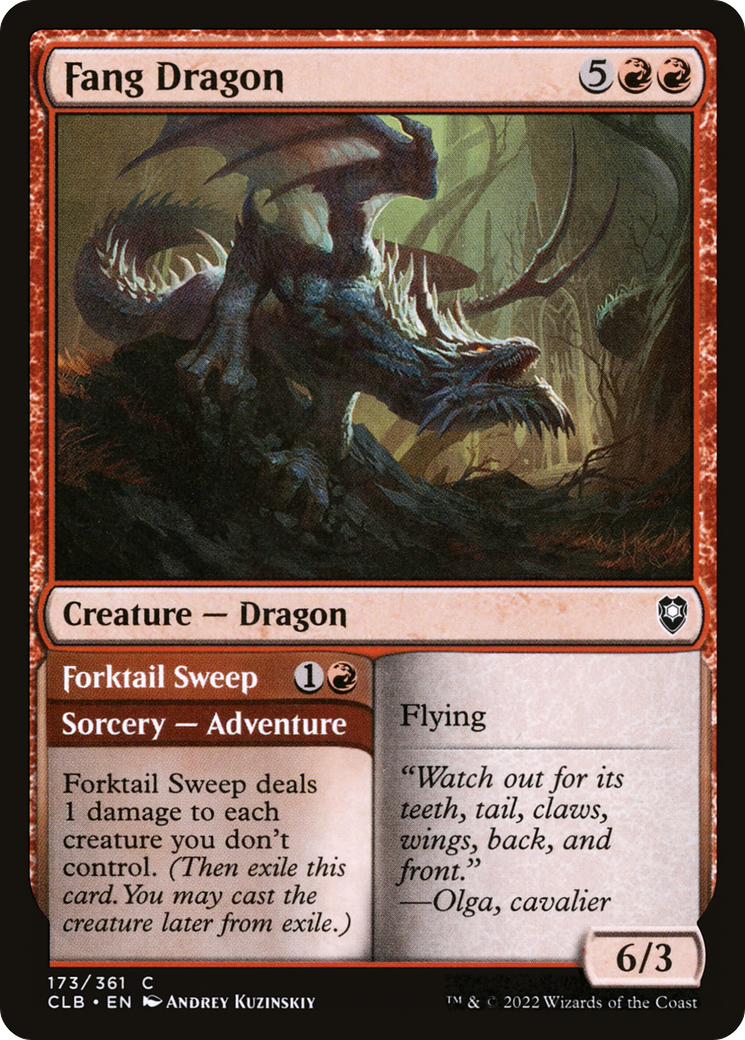This image depicts a trading card, likely used in a collectible card game. The card features a dramatic illustration of a "Fang Dragon" perched on a rock set in the bottom left of the card's top half. The dragon, with its menacing fangs, claws, wings, and long tail, dominates the center of the image. Surrounding it in the background are dark, brooding trees and hints of a building, adding depth to the fantasy setting. The title "Fang Dragon" is prominently displayed in black text at the top, followed by text that reads "Creature — Dragon." 

Below the illustration, the card details its abilities and effects: "Forktail Sweep" is a Sorcery Adventure spell that deals 1 damage to each creature the player doesn't control, and then exiles the card so the player may later cast the creature from exile. The card features a quote: "Fly and watch out for its Teeth-Tail Claws, Wings-Back-In-Front." The name Ogle Cavalier appears alongside this lore, contributing to the card's narrative richness. 

Additional details include a multicolored palette involving red, gray, green, yellow, and black. The card edges are black, and at the bottom, it reads: "Audrey Kosinski, 173361C, CLB.EN" on the left side, and "6/3, 2022, Wizards of the Coast" on the right, indicating its designer and publisher.